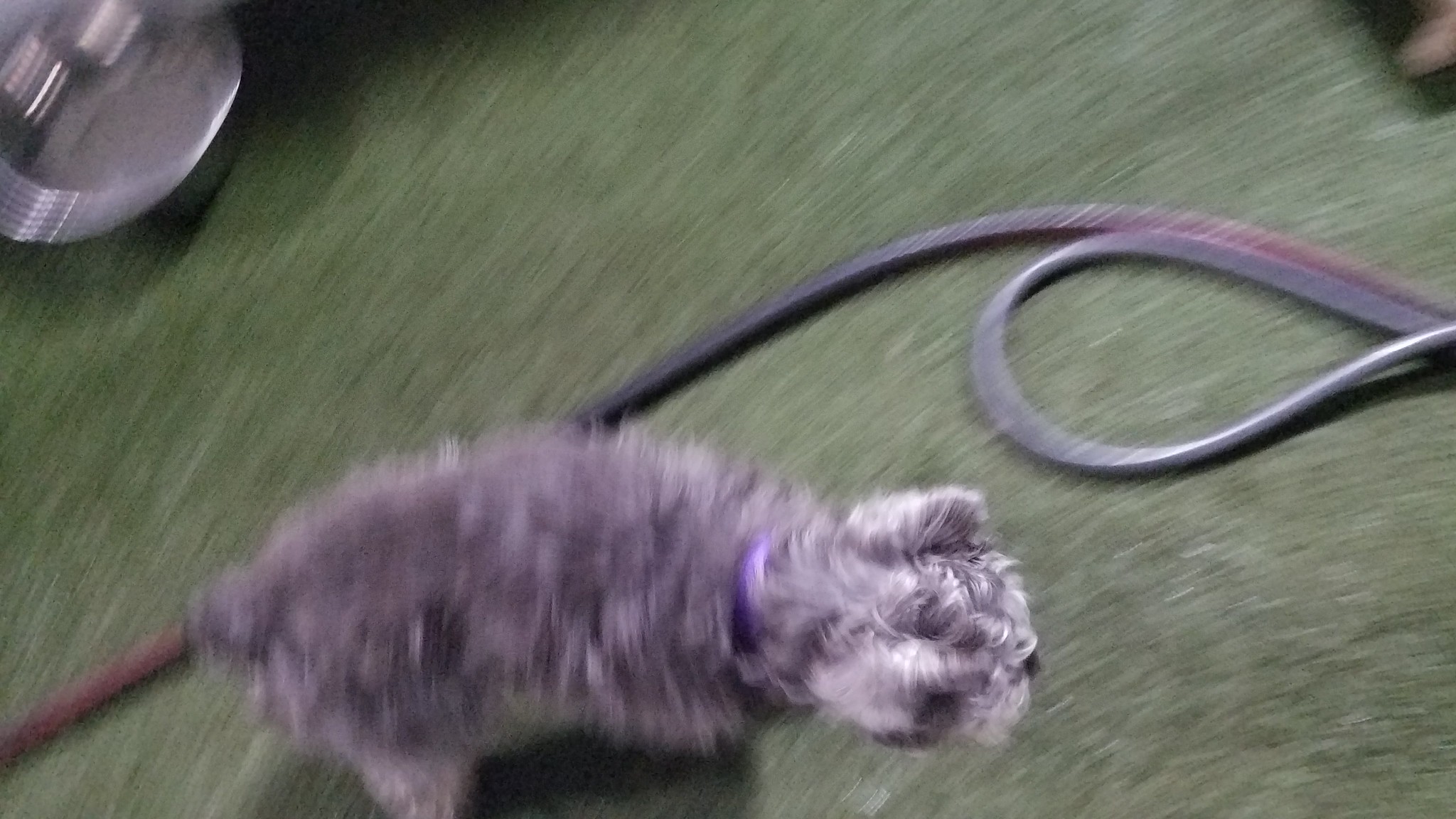This is a very blurry overhead photograph of a small gray terrier-like dog standing at the bottom center of the image. The dog has a scruffy, wiry coat with varying shades of gray and a purple collar around its neck. Its ears are perked up, and its little black nose points forward as it stands on a surface that appears to be either dark green carpet or grass, though the exact nature of the ground is obscured due to the blur. A thick black hose snakes across the center of the photo, looping from the bottom left to the right side. In the top left corner, there's a round, grayish, indistinct object, possibly metallic, and another blurry object occupies the top right corner. Despite the lack of clear detail, the primary focus remains the small gray dog, captured from above with its stubby tail and alert posture.